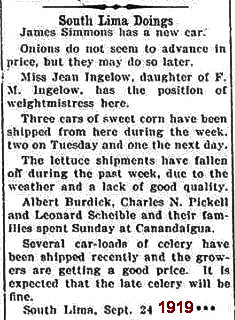This black-and-white newspaper clipping from September 24th, 1919, titled "South Lima Doings," features various local updates. It highlights that James Simmons has acquired a new car and notes that while onion prices have remained stable, an increase is possible. Ms. Jean Ingelo, daughter of F.M. Ingelo, has secured a position as wait mistress. The article also reports that three carloads of sweet corn were shipped out this week—two on Tuesday and one the following day. However, lettuce shipments have decreased due to poor weather and quality issues. Additionally, it mentions that Albert Burdick, Charles N. Pickle, and Leonard Scheibel, along with their families, spent Sunday in Canandaigua. It also notes that several carloads of celery have been shipped recently, with growers receiving good prices and high expectations for the late celery crop. The date is prominently displayed with "1919" in red followed by an ellipsis in black.